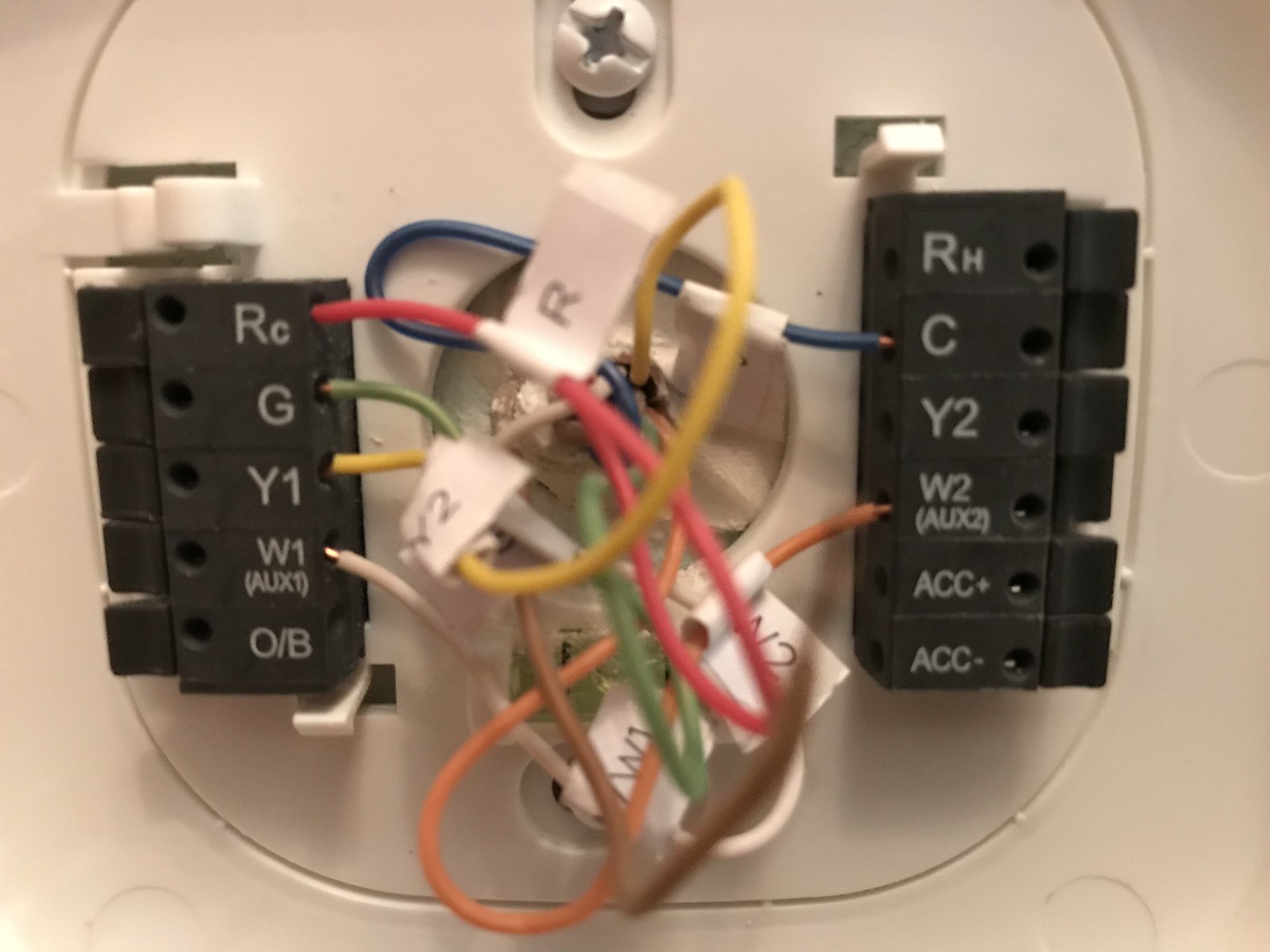This close-up image shows an electrical box embedded in a wall, featuring an array of tangled, multi-colored wires. Central to the image is a painted screw at the top center, securing a plastic plate. The box appears to be for a light switch or a similar fixture. 

On the left side of the box, labeled fuses read: RC, G, Y1, W1 (AUX1), and O/B. The wiring configuration reveals a red wire connected to RC, a green wire to G, a yellow wire to Y1, and an off-white wire to W1. Notably, the G, Y1, and W1 fuses are depressed, indicating they are active, while RC and O/B fuses are not depressed, suggesting they might be inactive.

On the right side, another set of fuses are labeled as R, H, C, Y2, W2 (AUX2), ACC+, and ACC-. A blue wire is connected to the C fuse, and an orange wire is connected to the W2 (AUX2) fuse. Both of these fuses are depressed, indicating live connections.

The image captures the intricate details of the wire connections and fuse arrangements, providing a clear view of the internal configurations of this electrical component.